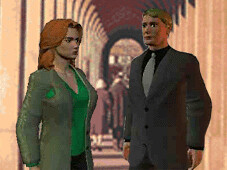This image appears to be a highly detailed screenshot from a video game. The foreground features two prominently positioned characters. The female character on the left is wearing a distinctive outfit consisting of an olive green jacket and a forest green shirt with an emerald logo. Her shirt has a v-neck that reveals part of her chest and neck. She has short, orange hair and a pale complexion, complemented by red lips and a stern expression. She is dressed in black pants. 

Opposite her, the male character on the right is taller, with darker skin and short, brown hair that could be described as dirty blonde. He is dressed in a formal black suit with a button-down front, a black undershirt, and a light gray tie, exuding an air of sophistication.

They stand in a walkway marked by several arches along the sides and rear. The hallway extends into the background, where two other figures are seen. One appears to be a female wearing a long coat with light-colored sections and either gray hair or a scarf. The other figure is too distant to clearly identify. The architecture includes pillars casting shadows, with a maroon red ceiling and a distinctly colored arch at the end of the hallway leading into a tan and light brown room. Overall, the characters have a stiff, almost mannequin-like appearance, giving the scene a surreal, doll-like quality.